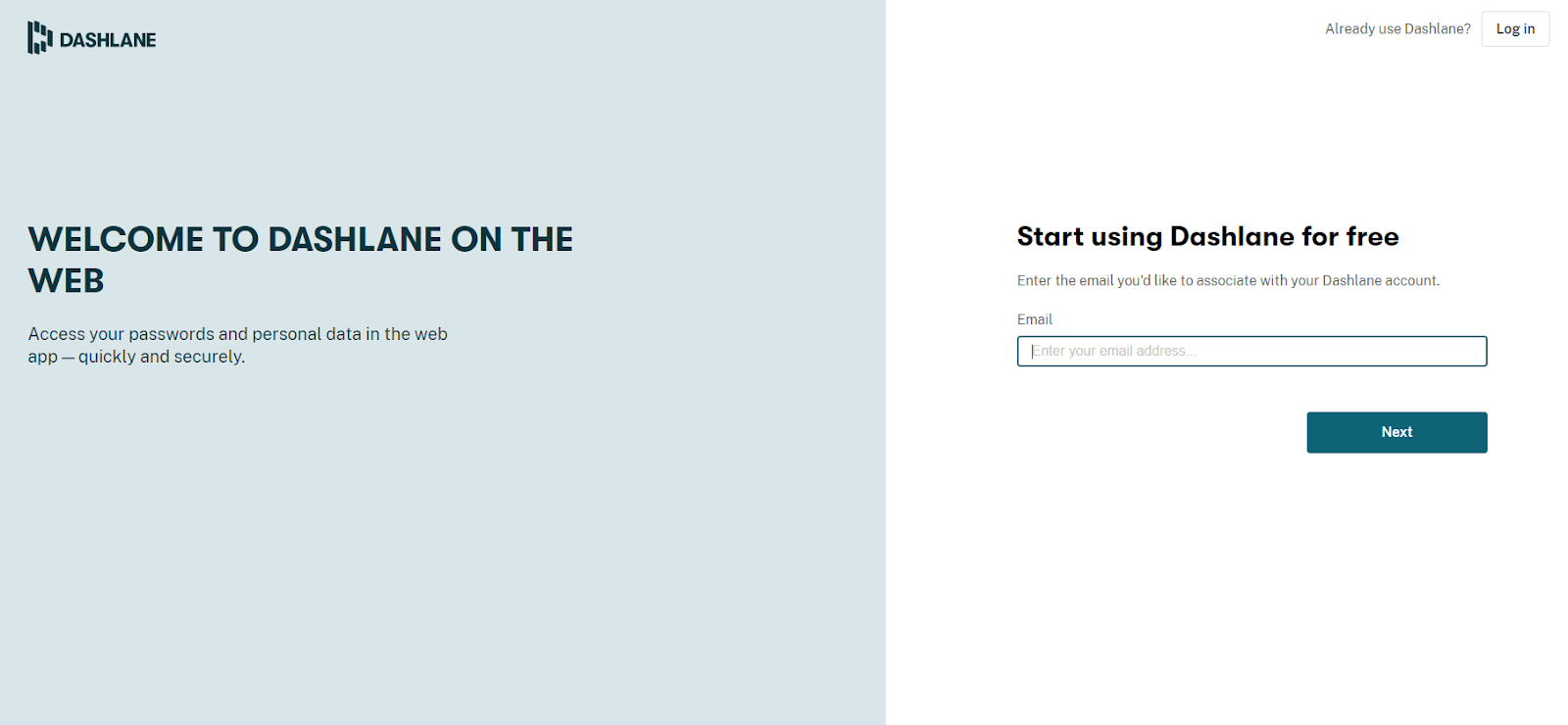The image displays a webpage from Dashlane, a password management service. The page layout is divided vertically, with the left side featuring a gray background and the right side in white. At the top of the page, the Dashlane logo is visible with a stylized 'D' made of block shapes.

In the center of the page, bold text reads "Welcome to Dashlane on the web," followed by a smaller black print that says, "Access your passwords and personal data in the web app quickly and securely." On the right side, there is a section for existing users with the prompt "Already use Dashlane?" accompanied by a rectangular login button.

Lower down the page, a section invites new users to start using Dashlane for free. It instructs visitors to "Enter the email you’d like to associate with your Dashlane account," followed by a field labeled "Email" with placeholder text that reads "Enter your email address...". Below this field is a button labeled "Next," which is dark teal or gray in color, with the word "Next" written in white.